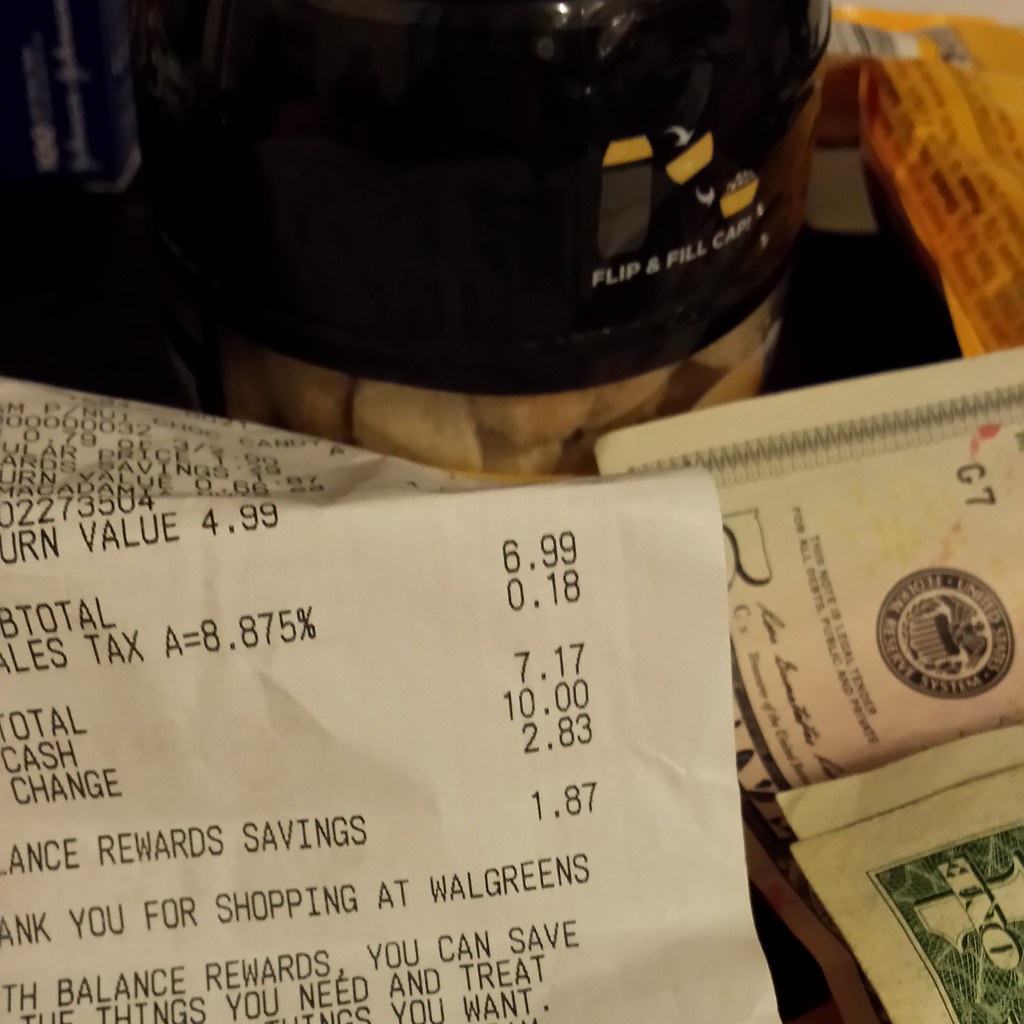The image shows a detailed snapshot of various items, with the focal points being a crinkled white receipt and a small collection of American currency. The receipt, positioned on the left side, is from Walgreens and contains several key details: a purchase total of $7.17, $10 in cash given, and $2.83 in change returned. The receipt also includes mentions of sales tax, which is calculated at 8.875%, and a partial message thanking the shopper for visiting Walgreens. Some of the text is faint and partially obscured due to its crinkled state. On the right side of the image, partially folded and slightly stained, are two $1 bills and one $5 bill in American currency. At the top of the image, there is a black object, identified as a coffee maker, featuring visible instructions that read "flip and fill cap." This coffee maker provides a practical backdrop to the scene.